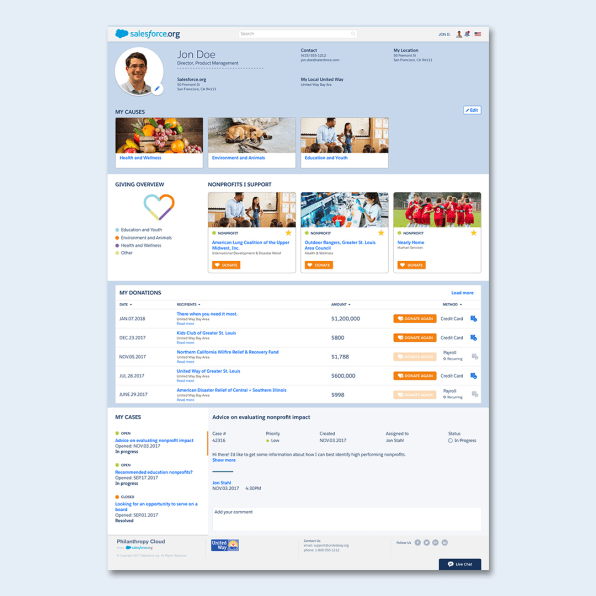This is a screenshot of the Salesforce.org website, specifically showcasing a user's profile page. The profile appears to be fake and is attributed to "John Doe," who is listed as the Director of Product Management. The page includes several sections such as "Contacts," although the phone number displayed is blurred and unreadable. Under the "My Causes" section, the user's interests include "Health and Wellness," "Environment," "Animal Welfare," "Education," and potentially "Truth" (the text is somewhat unclear). Additionally, there are sections titled "Giving Overview," "Nonprofits I Support," and "My Donations," which likely detail the user's philanthropic engagements and financial contributions.